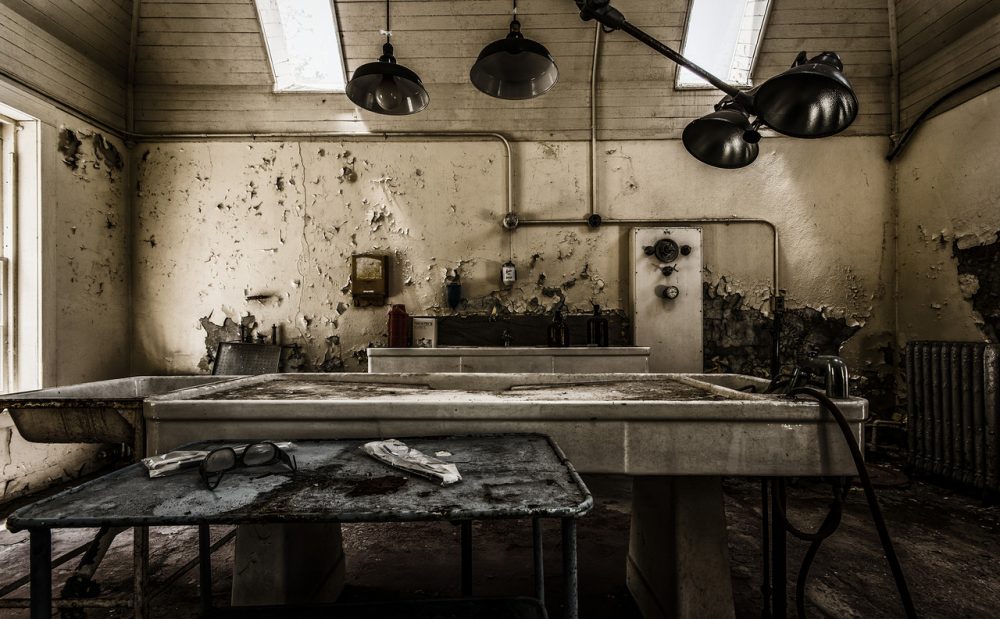The image depicts a massively dilapidated and grimy room that likely experienced a fire. The ceiling, made of beige or tan wood, features two rectangular skylights and is adorned with four black lights, none of which are illuminated. The walls are severely damaged, with peeling, cracked, and missing paint, giving the space a look of utter neglect. Pipes run along these marked and scratched walls, adding to the tarnished ambience. A dark black shelf stands at the back of the room, further accentuating the pervasive sense of decay.

In the foreground, there is a large, long rectangular table covered with dirt and garbage. In front of it, there is another table, black and seemingly burnt, which holds a pair of black glasses and a couple of pieces of paper, all enshrouded in filth. A rusty white chest is also situated near the back wall next to a big silver sink-like structure. The floor, covered in layers of dirt and debris, appears precarious and unstable, as if it could collapse at any moment. The entire scene is bathed in a palette of beiges, browns, and blacks, giving the room an eerie, abandoned feel, reminiscent of an old mortuary or a room where autopsies might have been performed.